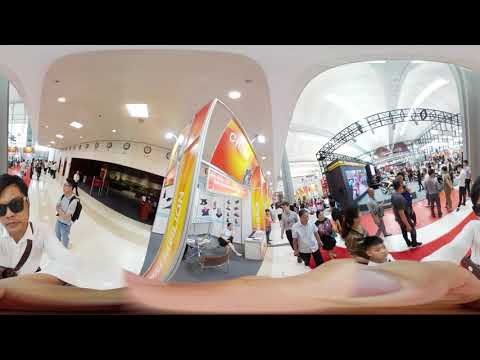The image depicts the bustling interior of a large, likely Asian, shopping mall where an event is taking place. The mall's architecture features predominantly white walls and tall ceilings adorned with bright lights, which give the space a vast and open feel. In the center of the frame sits a small stall or shop, possibly a shoe vendor, managed by one person. To the right, a significant stage setup complete with perimeter lighting suggests a concert or significant event is occurring, drawing a substantial crowd of onlookers. The crowd is diverse, including children, older individuals, and some wearing badges around their necks, indicating a mix of attendees. To the left, the mall extends into a long hallway lined with stores, although it appears less busy with relatively dim lighting. The overall impression is of a vibrant, crowded, and eventful section of the shopping mall.